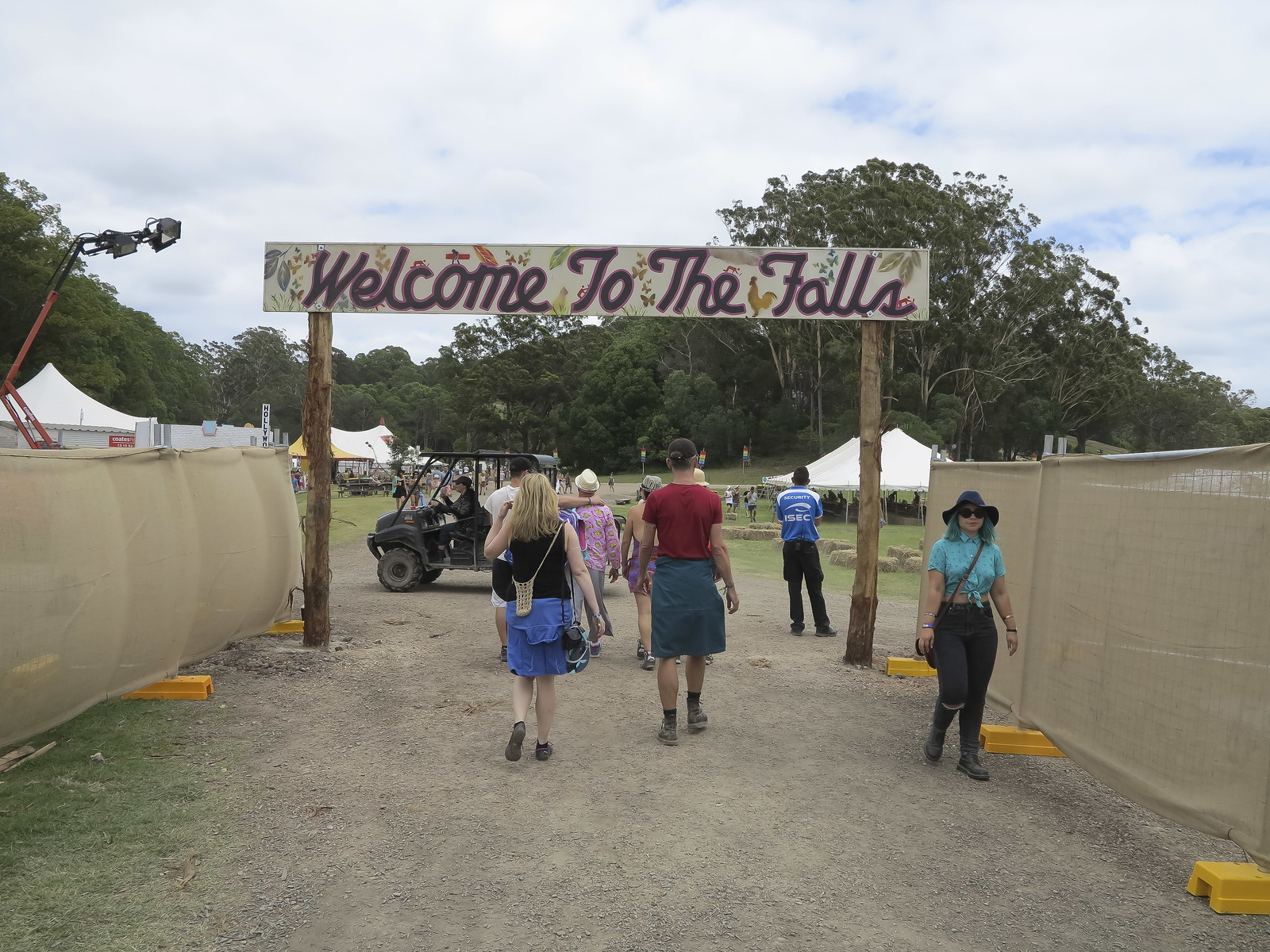The photograph depicts an entrance to a scenic area marked by two large, weathered wooden posts supporting a banner that reads "Welcome to the Falls" in purple font. A dirt path, bordered by makeshift fabric fencing and netting, leads towards the sign where several people, some wearing hats and casual attire, walk along. One notable woman in the foreground, dressed in a blue shirt, black pants, a hat, and carrying a purse, is walking away from the sign towards the camera. A four-wheeler is parked nearby, implying either security or transportation services. More background details include numerous canvas-like tents and canopies setup on either side of the path, along with hay bales and scattered lawn chairs. An additional vehicle equipped with an arm lift is visible near the tents. The scene is set against a backdrop of tall, thin trees under a mostly cloudy sky with slight blue patches peeking through, giving it a tranquil yet bustling outdoor fair ambiance.